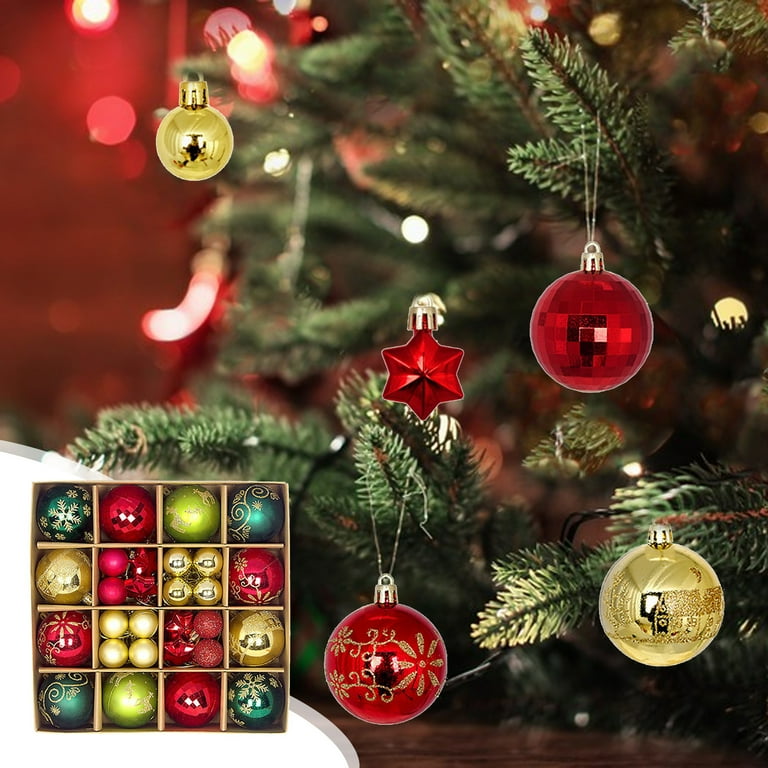This festive advertisement showcases a box of Christmas ornaments positioned in the lower left corner of the image. The box contains 16 individual compartments, each holding variously sized glass ornaments. The larger ornaments come in rich colors such as deep green, vibrant red, lime green, teal, and shimmering gold. The smaller ornaments, grouped in sets of four per section, exhibit a mix of festive hues. Notably, there is a small star ornament with a silver cap, a round red disco ball-themed ornament with a silver cap, a gold ornament adorned with glitter, and a red ornament featuring a snowflake motif with a silver cap. 

In the background, an artificial Christmas tree is prominently displayed, with the ornaments from the box digitally superimposed to appear as though they are hanging from its branches. The tree is subtly faded in some areas to draw attention to the intricate textures and designs of the ornaments. It is also illuminated with small, twinkling lights, enhancing the shiny glow of the ornaments. The composite image effectively emphasizes the variety and elegance of the ornament collection, making it ideal for a holiday advertisement.